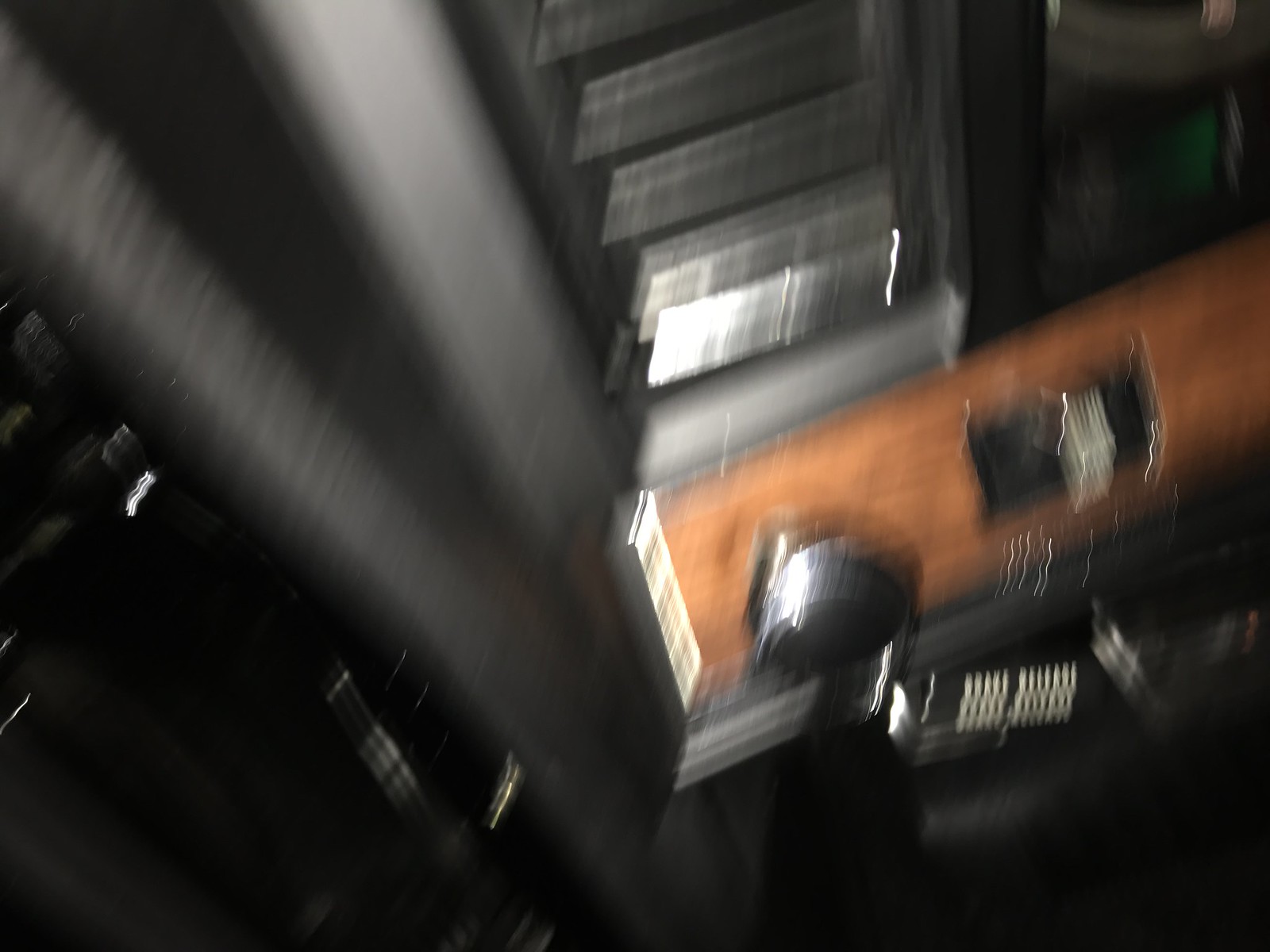The photograph appears to be taken in a landscape orientation and is heavily blurred, making the components difficult to distinguish. The image is dark and composed mostly of various shades of grey, along with some black, white, and brown hues. At the center-right of the image, there is a rectangular wood-grain panel with a medium brown or tan color, featuring chrome-colored edges. There are some mechanical and instrument-like elements within the scene. Notably, there is a dial on the left side of the wood panel and a switch to the right of it. Surrounding the panel, there are various black structures that are indistinct due to the blur. Additionally, a vertical chrome piece rises from the bottom center to the top left of the photo. In the distant background, a hint of green suggests the presence of either a shelf or a wall, though the poor resolution makes it hard to confirm. The setting seems to resemble the interior of a car, possibly showing a dashboard amidst the indistinguishable details.